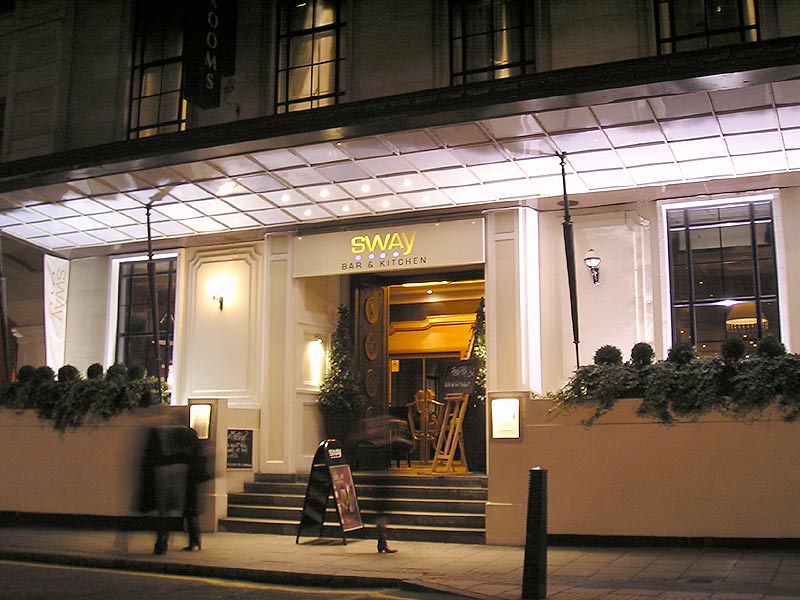The image is a color photograph taken at night, capturing the entrance to a restaurant named "Sway Bar and Kitchen" in landscape orientation. The building features a beige overhang above the entryway, displaying a gold-lit logo that reads "Sway" with "Bar and Kitchen" in smaller black letters below it. 

The entrance itself is highlighted by modern grid lighting and has double doors, partially open, inviting a glimpse inside. To access the entrance, visitors must ascend a series of five steps from the sidewalk. A sandwich board sign with a menu stands prominently at the base of the steps.

On either side of the entrance, large planters house meticulously trimmed topiaries and lush ivy, adding a touch of greenery. The scene includes two blurred figures walking by, suggesting movement caught in a long-exposure shot. The exterior also boasts expansive glass windows, but the inside of the restaurant remains hidden in the image. The overall ambiance is cozy yet sophisticated, enhanced by strategically placed wall lights.